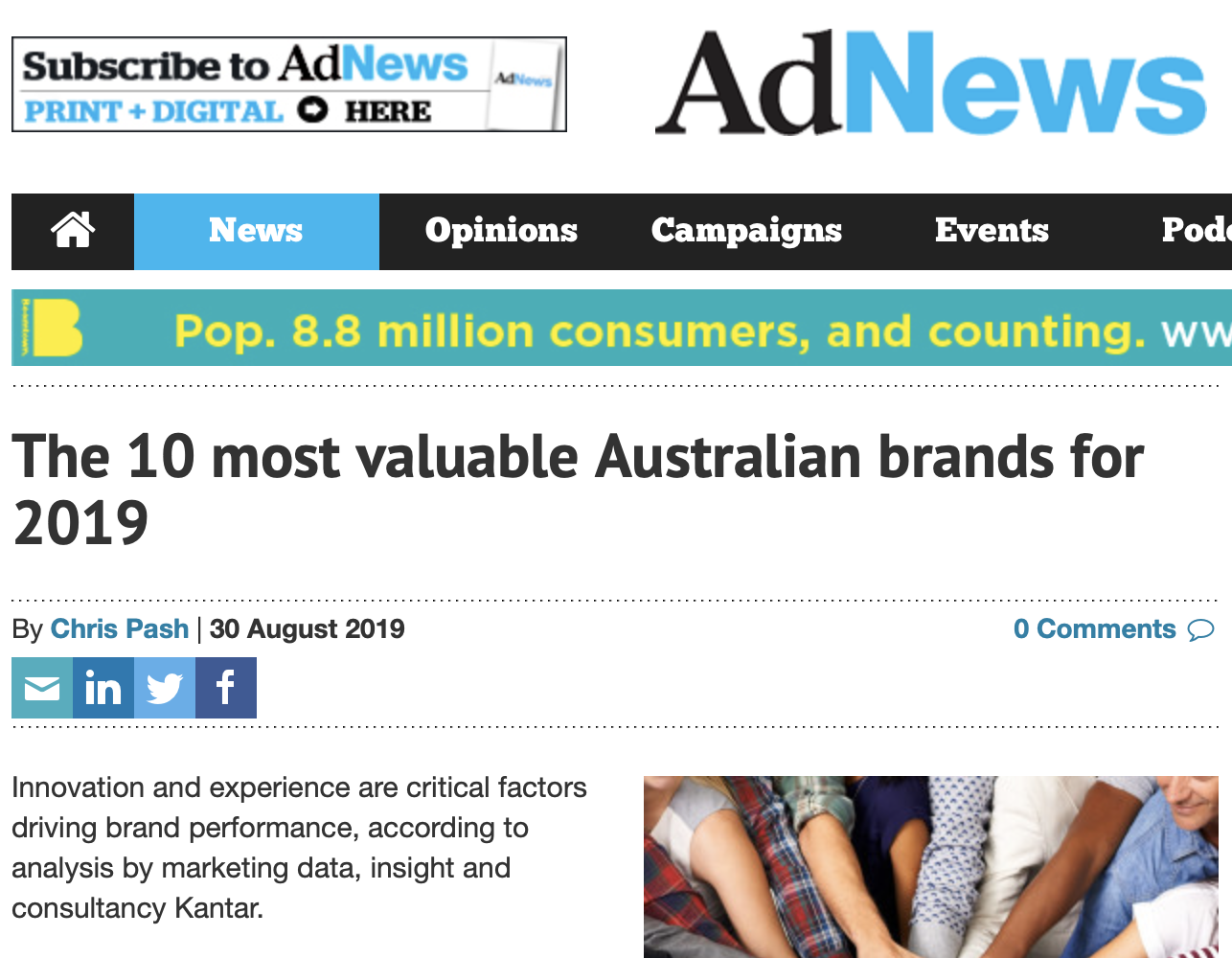This image resembles a digital article from an online newspaper platform named "Add News." The header prominently features the site's name, with "Add" (in black text) and "News" (in blue text). On the right side of the header, there is a prompt encouraging visitors to "Subscribe to Add News: Print and Digital."

Directly below the header, a navigation bar includes a series of menu items: "News," "Opinions," "Campaigns," "Events," and a partially truncated "Pod..." likely indicating "Podcast." The "News" section is highlighted in a blue box, indicating that it is the current selection.

Under the navigation bar, a bluish-green rectangle features a distinctive yellow capital "B" followed by some incomplete text: "Pop. 8.8 Million Consumers and Counting." It is cut off shortly after displaying: "WW."

The main article headline reads: "The 10 Most Valuable Australian Brands for 2019," authored by Krish Pash and dated 30 August 2019. It also indicates that there are zero comments on the article.

The accompanying image captures a group of people raising their arms collectively, suggesting a celebratory gesture or solidarity, as they prepare to take a group photograph.